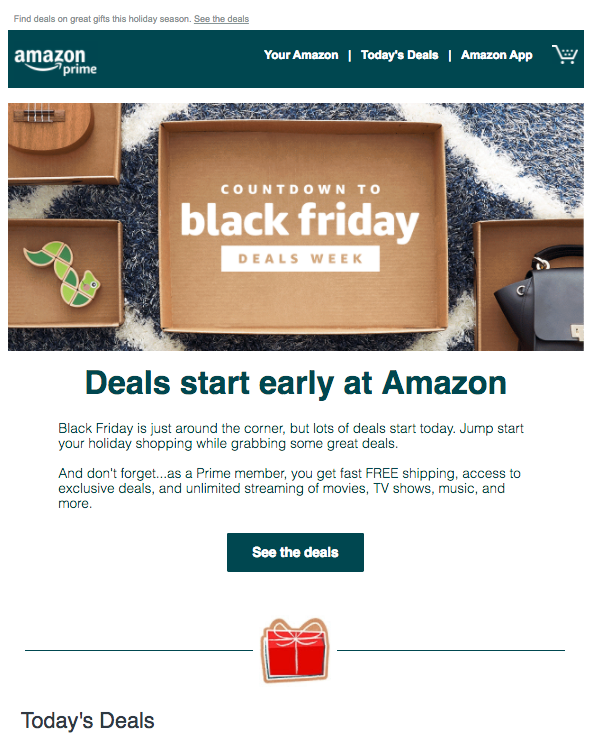The webpage appears to be a promotional section on Amazon's website, celebrating the Countdown to Black Friday Deals Week. The top of the page features a distinctive Amazon dark green navigation bar. On the left side of this bar is the familiar Amazon logo with an arrow underneath, followed by the word 'Prime'. To the right side of the bar, there are several clickable features including 'Your Amazon', separated by a vertical line from 'Today's Deals', followed by 'Amazon App', and a shopping cart icon.

Beneath the navigation bar is a large image occupying a significant portion of the page. This image showcases a brown box with text reading "Countdown to Black Friday Deals Week" on it. The box appears to be placed on a field that resembles astroturf with football field lines. The top part of the image displays various items, including what looks like the bottom of a guitar and other small items in boxes. On the right side of the image, there is a small purse or wallet inside another brown box.

Below this main promotional image, there is a prominent headline in black uppercase letters that reads, "Deals Start Early at Amazon." Below this headline are a couple of paragraphs with additional details about the deals. Following the text, there is a dark-colored call-to-action box that urges visitors to "See the deals." This box is flanked by a small red present icon emitting lines on both sides, symbolizing excitement or importance. At the bottom left, there is a link labeled "Today's Deals."